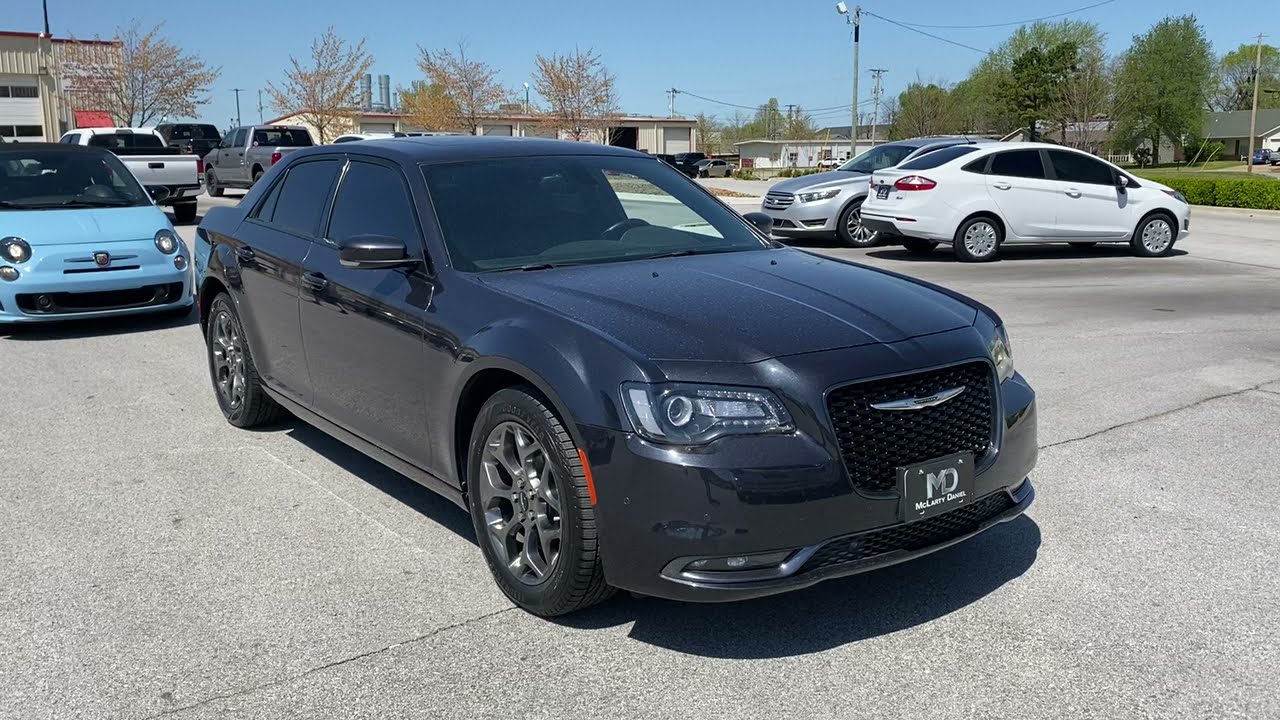In this detailed image of a parking lot taken midday, the center foreground showcases a prominent gray Genesis sedan and a small light blue Fiat, both positioned among several other parked and moving vehicles. The lot itself is paved with asphalt and shows visible cracks. Surrounding these central cars, a variety of other vehicles include a white pickup truck, a black truck, and a gray truck towards the back of the parking lot. On the right side, a white car faces the road and a gray Audi faces inward. 

The background reveals a mix of industrial and residential features, including older buildings with smokestacks, perhaps indicating a factory. Just behind these structures stands a large tan building with multiple white roll-up garage doors, one of which is open. Further to the right, you can spot a trailer and a couple of houses enveloped by green grassy lawns and evergreen trees. A series of power lines is also discernible in the distance.

The sky above is a clear blue, adding a crisp contrast to the colors below—grays, whites, blues, browns, blacks, tans, and reds. There is no text visible anywhere in the image. Overall, the image captures an everyday outdoor parking lot scene with a variety of cars and background details, providing a sense of a typical bustling yet organized space.